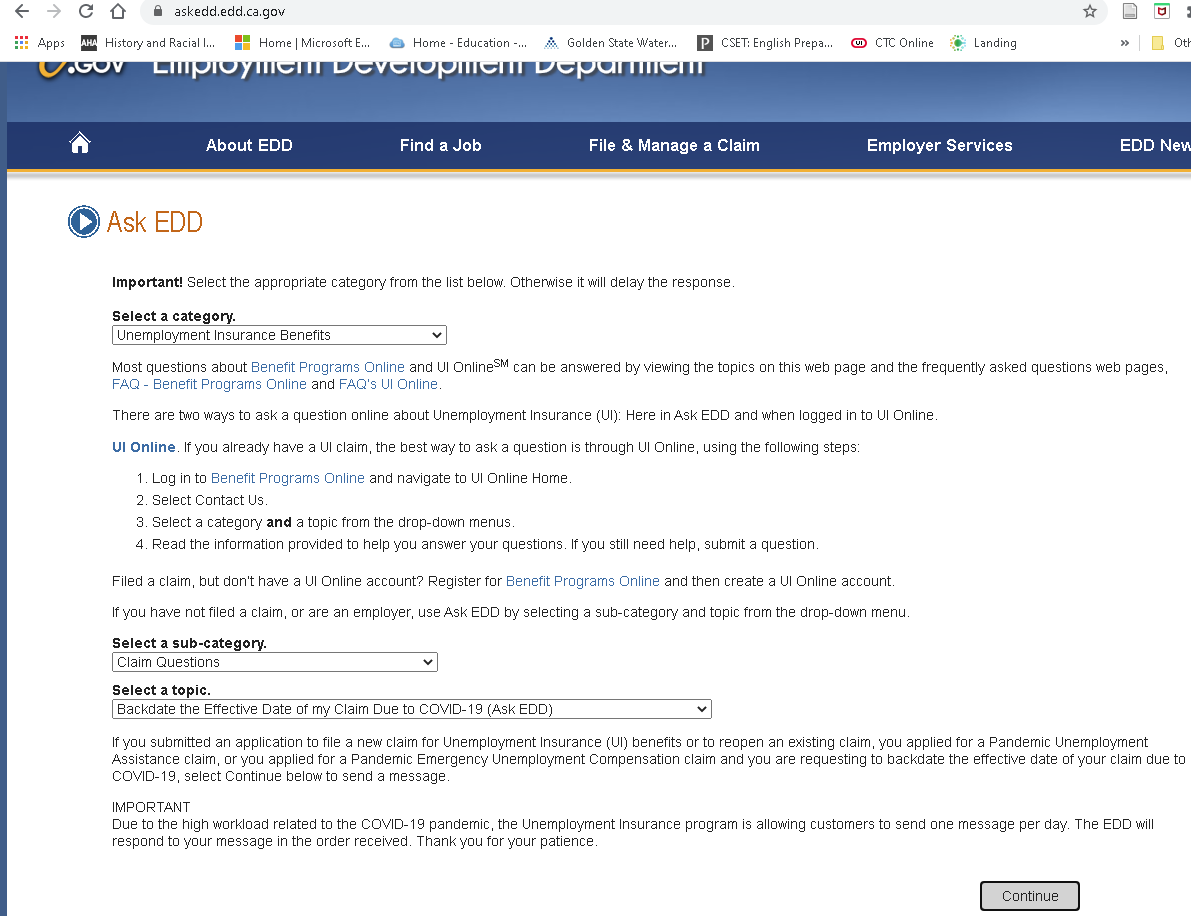This image displays a detailed partial screen capture of a web browser viewing a specific website. The browser's interface is visible at the top, featuring standard navigation buttons like forward, backward, reload, and home, along with a URL entry bar. A lock icon indicates the site is secure. Various other functional icons are also present. Below this, a secondary row of icons and options are shown.

The main content of the capture is a website, predominantly outlined in blue and white. At the top, a blue bar prominently labels the site as the "Employment Development Department." Directly below this, another blue navigation bar offers several options: Home, About EDD, Find a Job, File and Maintain a Claim, Employer Services, and EDD News.

The section beneath these bars features a white background and is titled "AskEDD" at the top. The main instructions inform users: "Important: Select the appropriate category from the list below, otherwise it will delay response." Below this instruction is a drop-down menu labeled "Select Category," allowing users to choose from various categories. Following the drop-down menu, there are several clickable text areas that provide more details about each category.

Further down, a second drop-down menu, "Select Subcategory," appears, allowing users to narrow down their selection. Additionally, there is another drop-down menu labeled "Select a Topic," which subdivides selections even further.

At the very bottom of the webpage, a "Continue" button is present, inviting users to advance to the next step after making their selections. The detailed layout and multiple drop-down menus suggest a structured and user-guided process for navigating the Employment Development Department's resources.